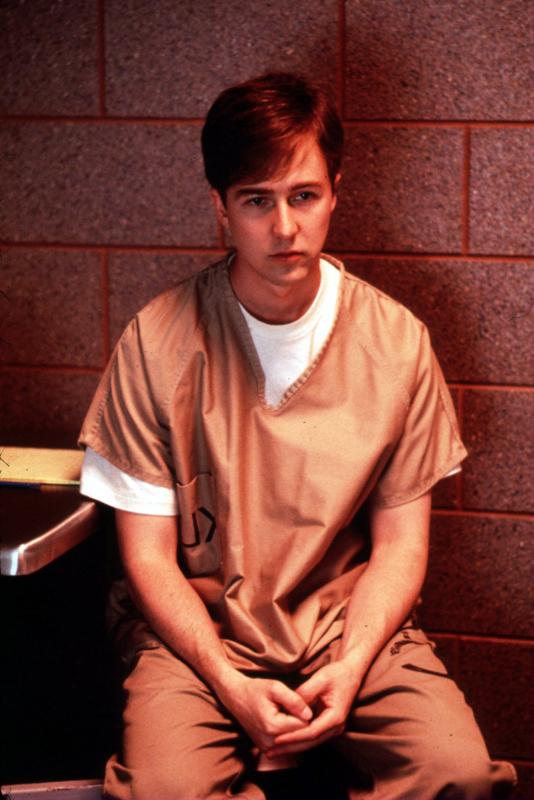This is a photo of a young actor dressed in prison uniform, sitting on a bench next to a partial view of a stainless steel table. Behind him is a wall constructed of burgundy-colored cinder blocks that cast a reflective glow, imparting a hint of burgundy to his short, dark hair, which is parted on the left and includes bangs. He wears a white t-shirt under the uniform and the colors in the photo exhibit a goldish, sepia, or orange-brown hue, enhancing the overall warm tones. His slender face, marked by a larger nose, shows no smile as he sits with his hands in his lap, thumbs crossed over one another. The deep, reflective tones of the wall contribute to the intense ambiance of the setting.